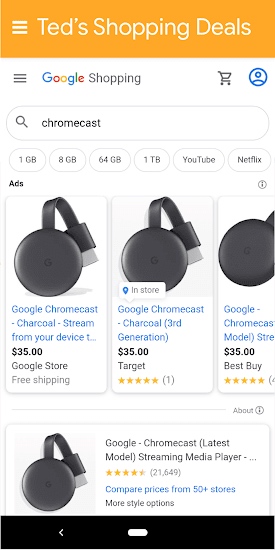This screenshot displays the shopping search results on a mobile device. At the top is an orange header featuring a white icon of three horizontal lines, commonly representing a menu, followed by large white text reading "TED'S SHOPPING DEALS." Below this header, the main portion of the page is set against a white background.

At the top left, there are three medium-gray, horizontally stacked lines, indicative of a menu. Adjacent to this, the Google logo is prominently displayed, with the letters in their iconic colors: blue, red, yellow, blue, green, and red. To the right of the Google logo is the word "SHOPPING" written in gray text. On the far right, the page includes a medium gray shopping cart icon and a blue, generic profile picture icon designed with white negative space.

Directly beneath this, a rectangular search bar with rounded ends features a medium-gray magnifying glass icon on the left and black text on the right stating "CHROMECAST." Below the search bar, there are several filter options displayed as rectangular buttons with rounded edges and gray text, listing "1GB," "8GB," "64GB," "1TB," "YouTube," and "Netflix."

Further down, a row includes the bold word "ADDS" on the left and an icon of a medium-gray eye encircled by a matching donut shape on the right. Following this row, three products are presented side by side. Each product is enclosed in a white rectangle with rounded corners casting subtle light gray shadows. The product listings feature images, blue product titles, bolded black prices, and thin black text indicating the store, accompanied by varying additional information specific to each item.